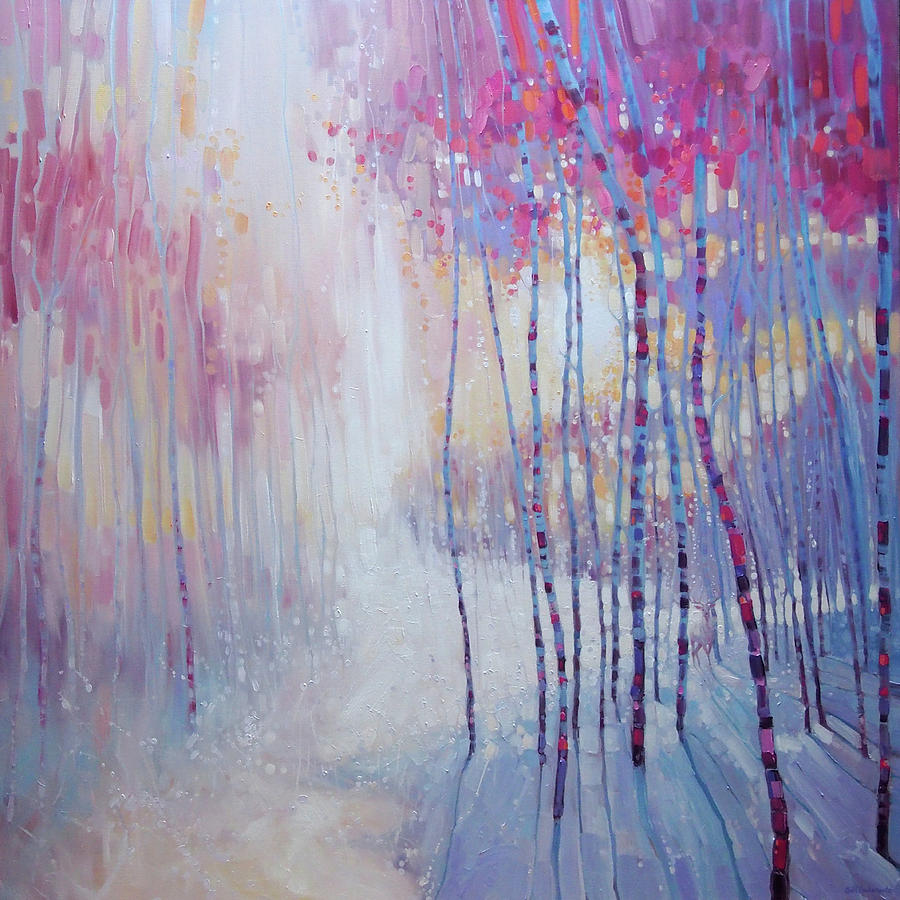This oil painting captures a snowy forest scene characterized by exceptionally tall, slender trees that stretch high above the viewer's perspective. The trees, with an almost misleading appearance of thin, elongated trunks, display a unique blend of colors. Their bases are adorned with shades of blue, pink, and purple, while their leaves burst into vibrant hues of green, orange, blue, yellow, red, and light pink at the top. This forest features a delicate, translucent aesthetic, reminiscent of both watercolor and oil painting techniques, which blurs some of the details, especially on the left side where the trees appear blurry and out-of-focus, almost creating an ethereal feel. The sky above transitions through orange and white tones, contributing a warm glow that contrasts with the cold, snowy ground. The ground itself is covered with a thin layer of snow, blending into a grayish-blue hue, with hints of a khaki-tan path winding between the trees. The tree trunks, with their ring-like patterns of white, red, orange, and black, resemble the coloration of a coral snake, adding an exotic touch to the wintry landscape. The rich texture and layered colors come together to create a mesmerizing, dreamlike portrayal of a serene winter forest.